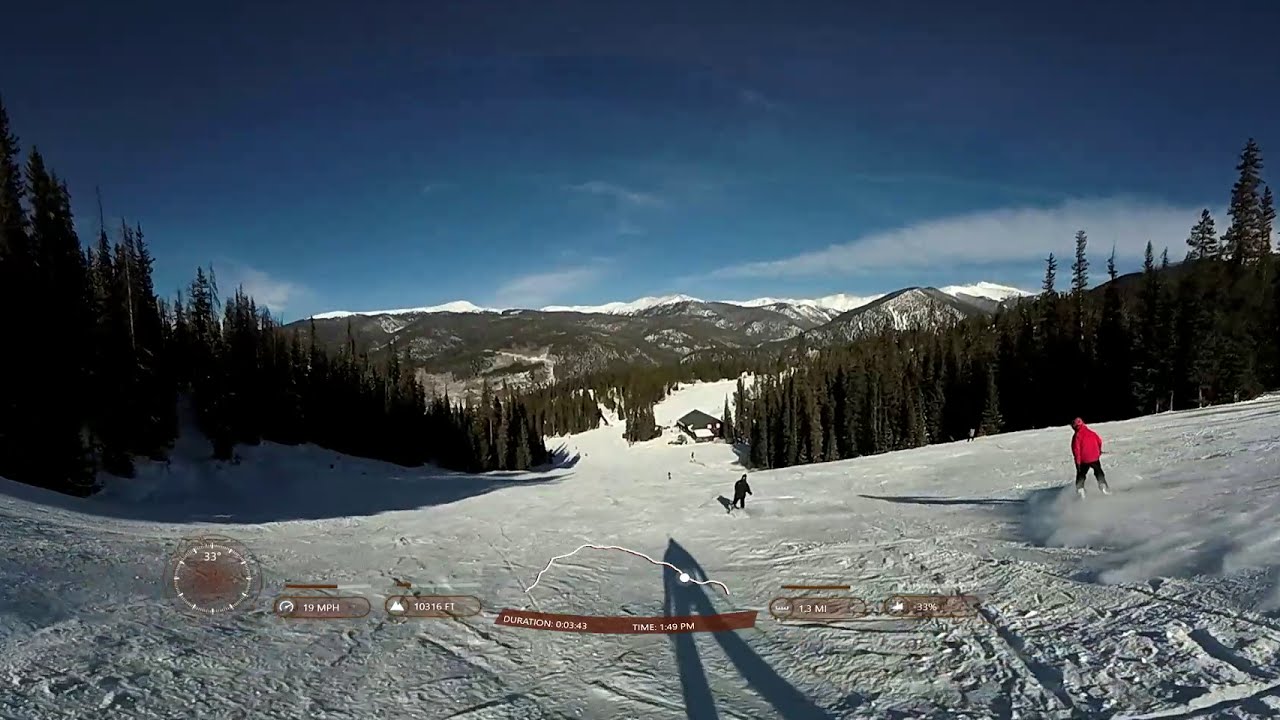The photograph captures a skier's point of view as they descend a snowy slope surrounded by dense, green pine trees. The upper part of the image features a light blue sky with white clouds, under which stretches a vast mountain range blanketed in snow. Midway up the image, snow-covered peaks dominate the background, providing a majestic, wintry vista. The slope itself is highlighted by patches of sunlight, emphasizing the crisp, clear conditions of the daytime setting.

The skier's shadow is visible at the bottom center of the image, showing the individual holding ski poles in both hands and wearing skis. Several other skiers can be seen further down, including a person in a red jacket, black pants, and white boots to the far right, and others dressed in darker clothing. There appears to be a ski lodge or small house at the base of the slope, adding to the bustling atmosphere of the scene.

An array of digital data overlays the bottom of the image, possibly from a HUD or smart device. This includes a speedometer reading 19 mph, an elevation of 10,316 feet, a time of 1:49 p.m., a duration of 0:03:43, and a distance of 1.3 miles. There is also a graphical progress indicator showing 33% completion of a route, providing real-time metrics for the skier’s experience.